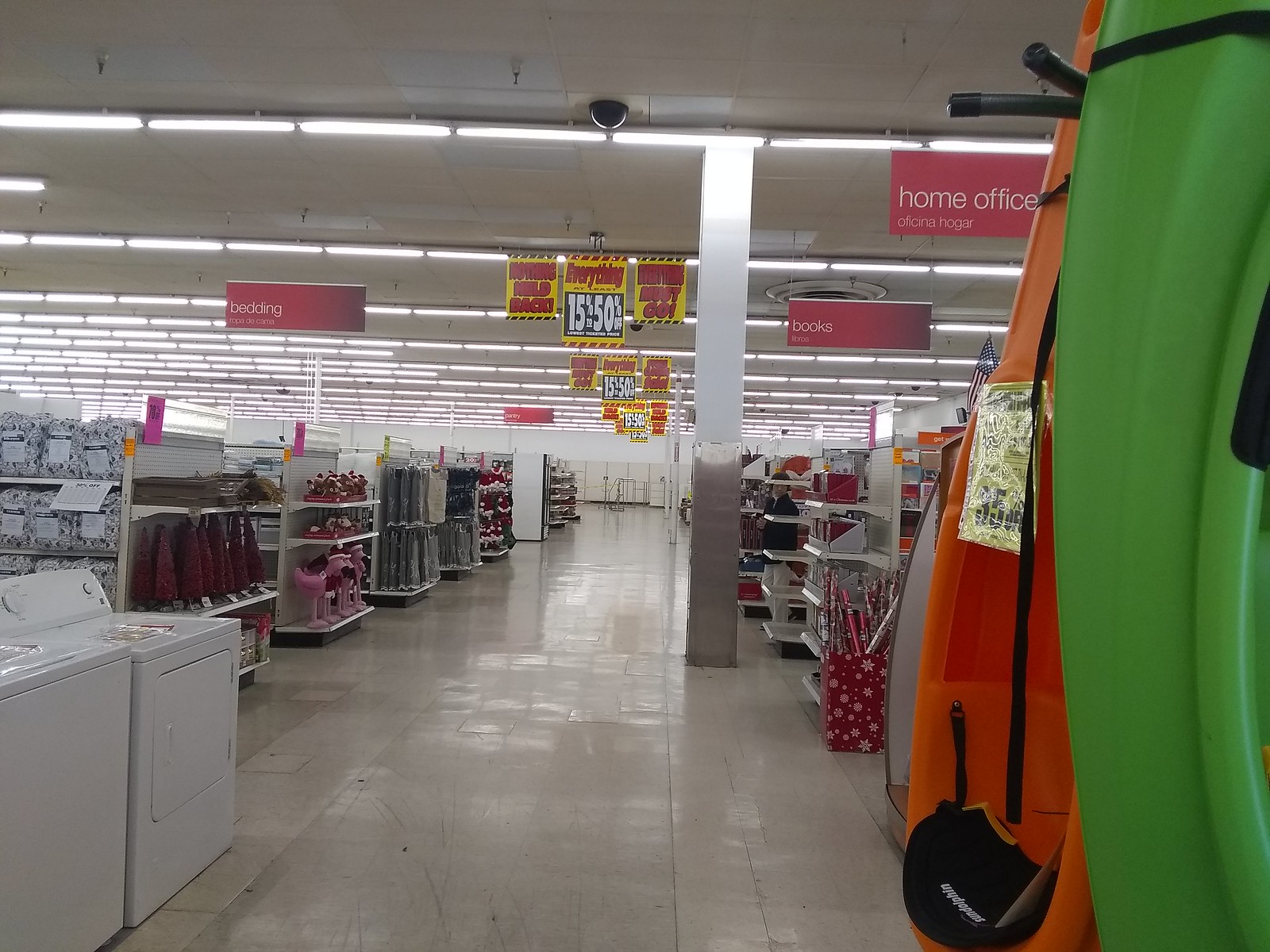In the image, there is an expansive department store with a glossy linoleum tile floor that reflects the bright overhead lights. The ceiling is tiled and adorned with multiple fixtures that emit a brilliant light, illuminating the entire space uniformly. Prominently, a white pillar can be seen supporting the ceiling. Hanging from the ceiling are various red signs indicating different sections of the store, such as "Books" on the right, "Bedding" on the left, and "Home Office" also on the right. Additionally, yellow signs are visible, advertising discounts ranging from 15-52%.

In the foreground, to the right, an orange kayak and a green kayak are displayed prominently. On the left, there is a washer and dryer set. The store is also stocked with numerous shelves filled with a wide array of products, making it an eclectic showcase of items available for purchase.